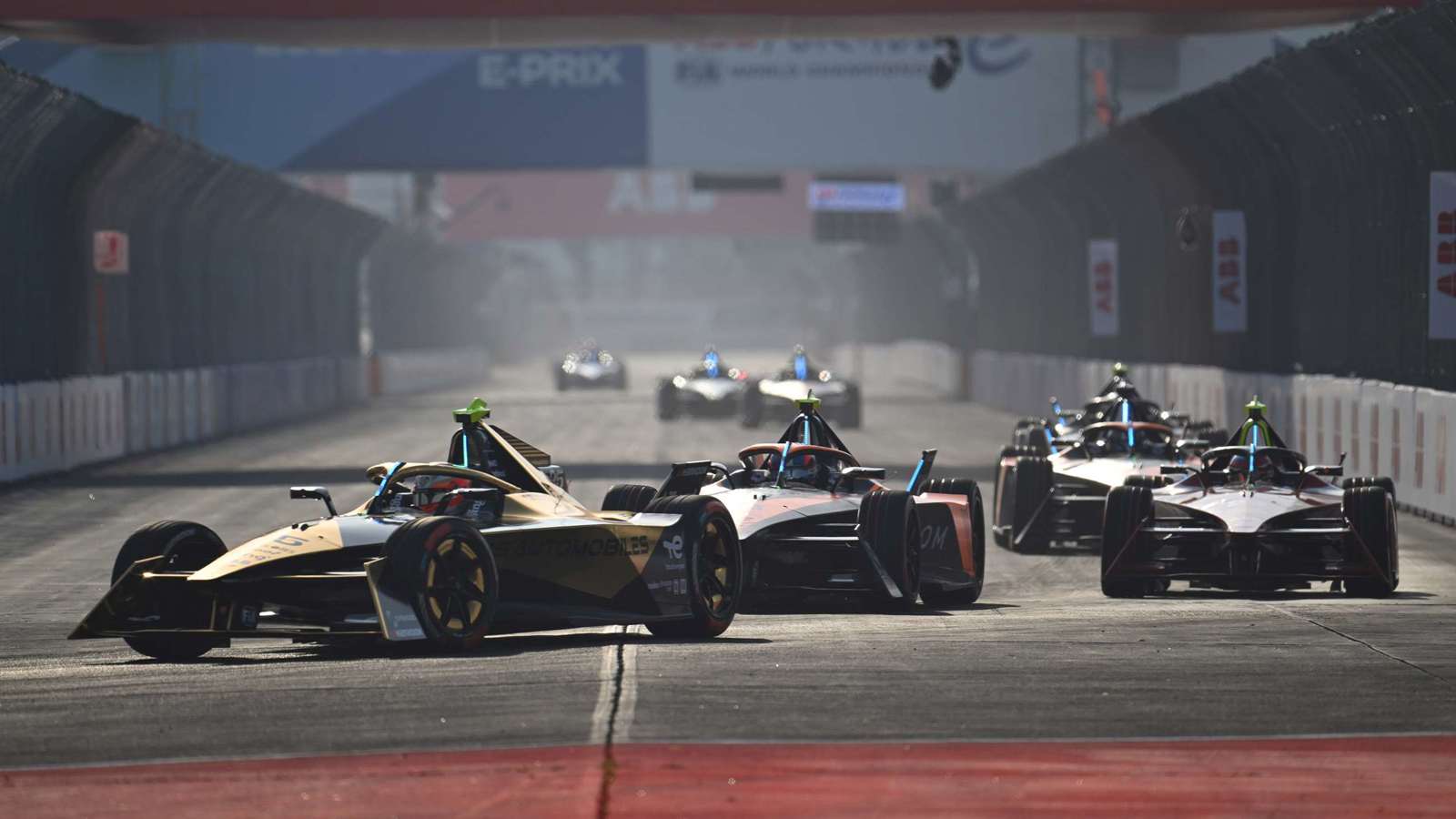The photograph captures a dynamic scene at a racetrack, where multiple sleek, single-driver race cars with open cockpits and large, oversized tires are speeding towards the viewer. The image is in a rectangular landscape orientation, with the width twice as long as the height. The racetrack, covered in gray asphalt, runs straight down the center of the image, gradually curving toward the left in the foreground. On both the left and right sides, there are tall walls featuring thick white barricades at the bottom and dark blue metallic panels above, with curved tops. A large, partially visible billboard spans the background, reading "E-Prix" in white text on a blue background, while the rest of the text is blurry and cut off.

Four cars dominate the foreground, with the leading car boasting a striking yellow and black color scheme. Just behind it, another car features a reddish or orange hue, and a third appears to have a green design. Additional cars are visible in the distance but become increasingly out-of-focus. The scene is imbued with the excitement and realism of competitive racing, capturing the intensity and intricacies of the sport.